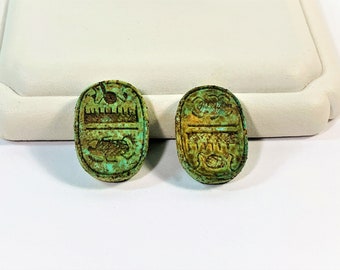This image showcases two small, ancient, oval-shaped metal artifacts resting on a white tabletop against a white velvet background, likely in a professional studio setting. The objects, possibly made of copper or a copper alloy due to their greenish and slightly brown oxidized patina, appear historically significant and are perhaps thousands of years old. Unrestored and dirty, these metal items feature intricate engravings and artistic drawings that are not clearly discernible because of the heavy oxidation. The artifacts, possibly dug up, resemble jewelry such as earrings or brooches, although they might also be belt buckles due to their indented tops. Despite their uncertain function, they're displayed prominently to focus attention on their worn, ancient beauty.